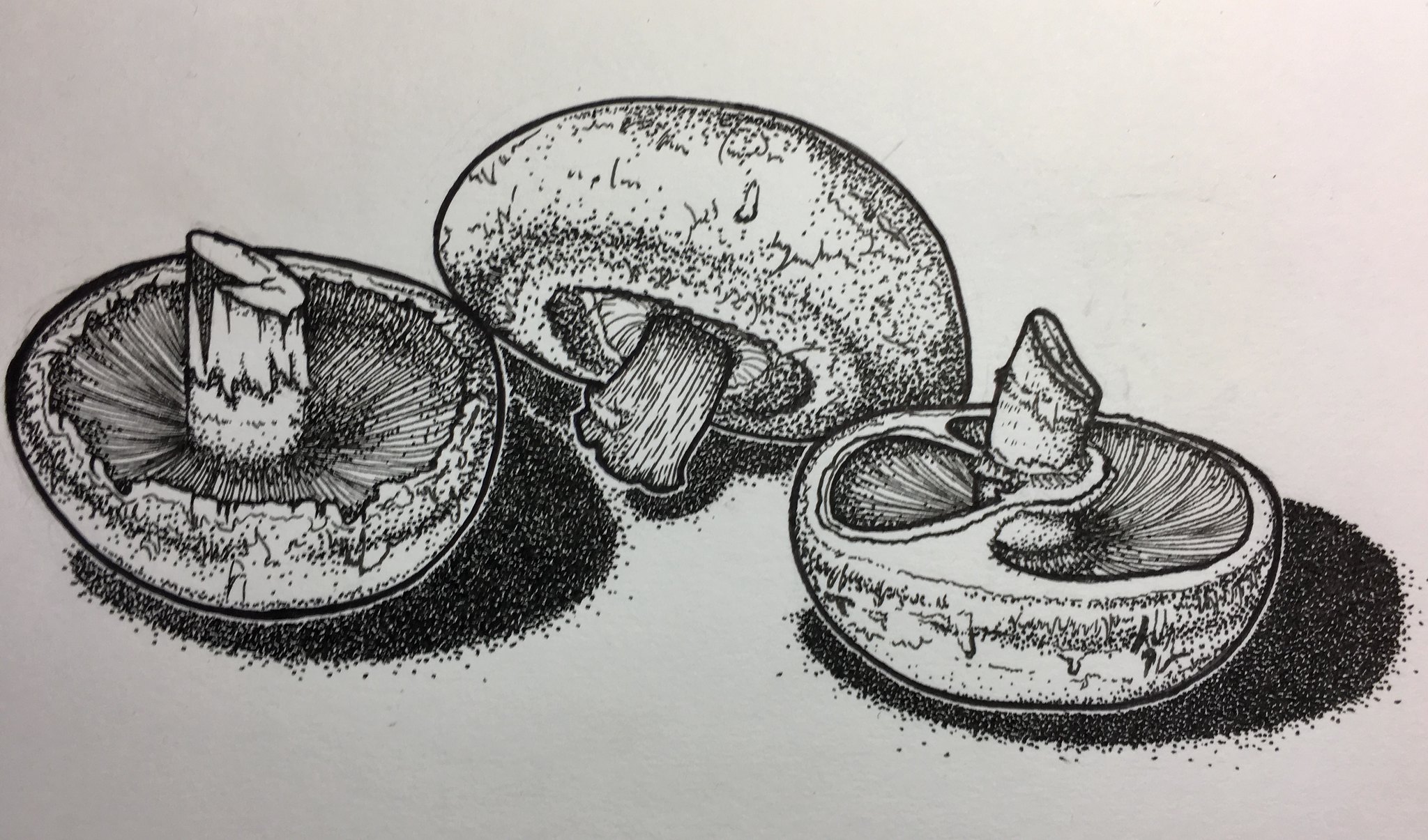This is a detailed black ink drawing of three button mushrooms on a very pale, possibly lavender-tinted, background. The mushrooms are arranged horizontal to each other. The central mushroom is laying on its side with its cap up and stem partially down, while the mushrooms on the left and right are upside down with their stems pointed upward. The artist has skillfully used pointillism to create detailed shading with black dots, giving texture to the mushroom stems and caps and creating shadows beneath each mushroom. The drawing captures the intricate lines of the gills and texture of the stems, making the mushrooms appear almost lifelike. The clustered arrangement of the mushrooms dominates the frame, showcasing the artist's detailed work against the pale background.